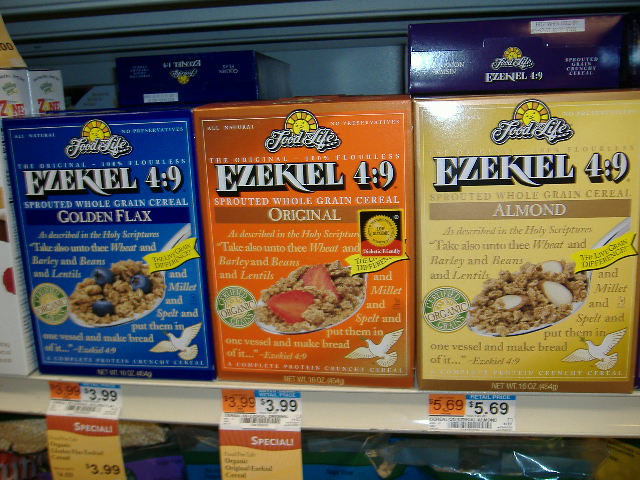The image depicts a close-up of a grocery store shelf displaying three different boxes of Ezekiel 4:9 Sprouted Whole Grain Cereal, each under the "Food for Life" brand with its logo displayed as an artsy, cartoonish sun. From left to right, the boxes are arranged in distinct colors: blue, orange, and yellow-golden. The blue box, labeled "Golden Flax," features an image of a spoonful of cereal with blueberries, matching the color of the box. The middle orange box, labeled "Original," showcases a spoonful of cereal accompanied by strawberries, reflecting the box's hue. The rightmost box is yellow-golden and labeled "Almond," depicting a spoonful of cereal with almond slices. Price tags beneath the boxes indicate that the "Golden Flax" and "Original" versions are priced at $3.99 each, while the "Almond" variant is priced at $5.69. The shelf itself is gray with a white front showcasing the prices.